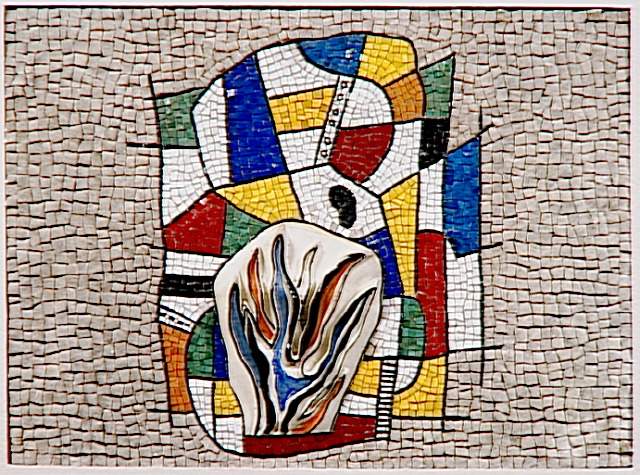The image depicts a detailed mosaic artwork composed of numerous small, unevenly shaped tiles. The primary background consists of light tan and off-white tiles that create a simplistic yet textured canvas. At the heart of this mosaic is a rectangle teeming with a vibrant array of tiles in various colors including green, white, red, yellow, blue, orange, black, and gold. These central tiles are arranged in a chaotic, almost primitive stained-glass fashion, bordered by visible spaces without grout. Dominating the center is an abstract, bulb-like figure, from which ornate, flame-like shapes in blues, reds, and blacks appear to emanate upwards, providing a striking focal point amidst the multicolored tile fragments.